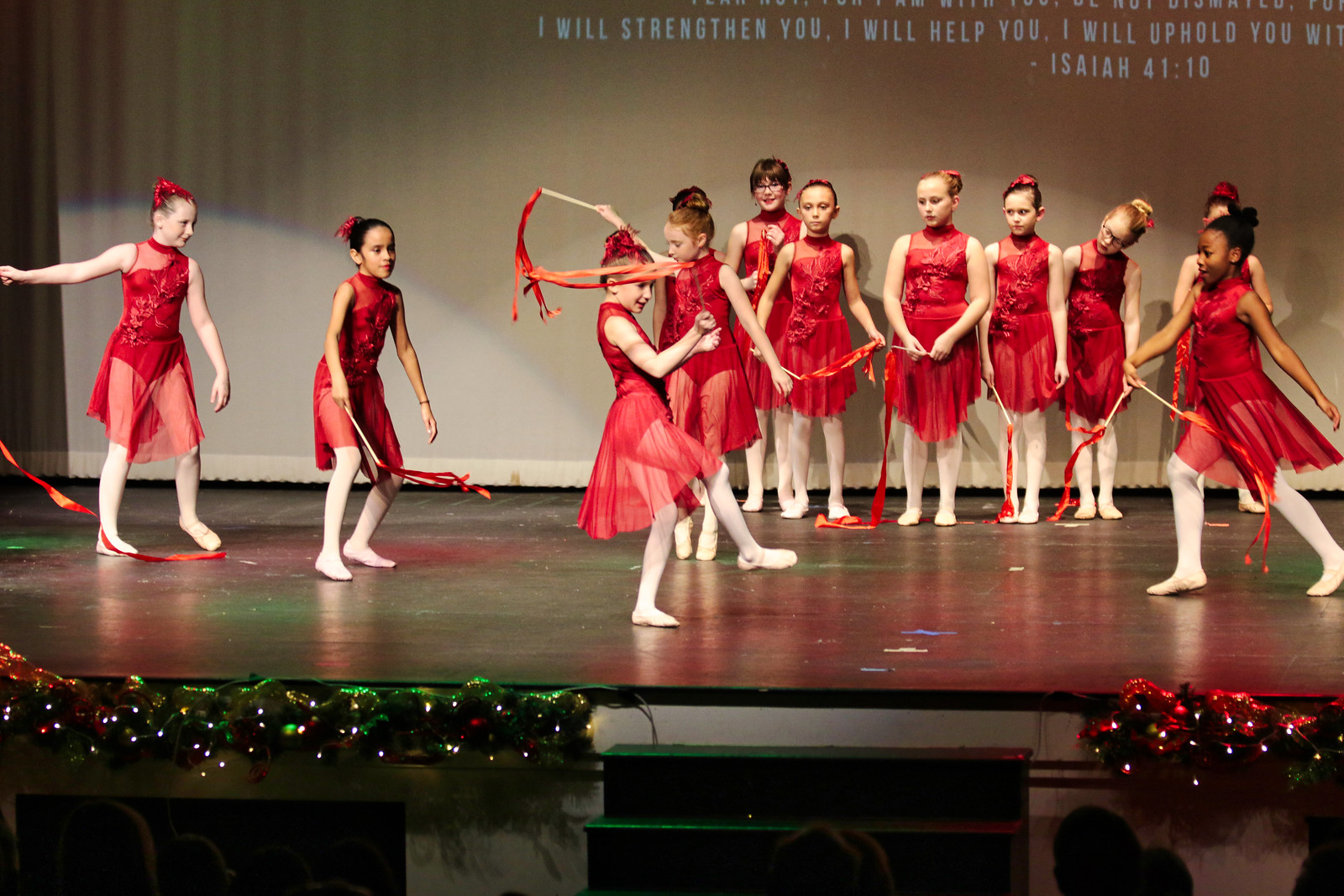The image is a landscape-oriented, color photograph featuring a mid-performance shot of about ten young girls, presumably 8 to 10 years old, dancing on a wooden stage inside an auditorium. They are dressed in matching red dance dresses with sheer skirts from the waist down, complemented by red bodysuits beneath. Red tights cover their legs, and their hair is neatly styled in buns wrapped with red ribbons. The girls are holding white sticks with red ribbons, which they are twirling. The stage has a grayish-tan backdrop, and a partially visible scripture is projected onto it, which reads, "I will strengthen you, I will help you, I will uphold you. Isaiah 41:10." The scene is framed with festive Christmas decorations, including greenery adorned with red and green fairy lights at the front of the stage. In the foreground, one girl, who appears to be a featured dancer, is facing to the right with her leg lifted. The dark auditorium reveals the silhouettes of audience members watching the performance, adding to the intimate and festive atmosphere of what likely is a church Christmas concert.